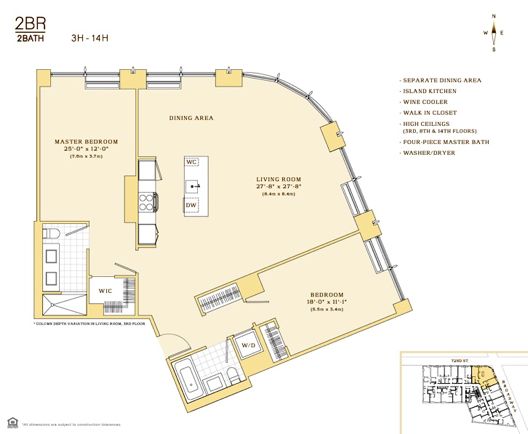A professionally drafted floor plan of a two-bedroom, two-bathroom apartment reveals a unique corner layout, utilizing the building's edge to create an open, wedge-shaped central space. The upper right-hand corner notes the "2BR2Bath" format.

The left side of the plan designates the Master Bedroom, featuring an en-suite bathroom with a toilet, dual sinks, and a shower (though initially mistook for a tub). This bedroom also includes a spacious walk-in closet equipped with racks for hanging clothes and a generous bed area.

On the opposite side, the second bedroom offers a smaller bathroom with a toilet, single sink, and a bathtub. Instead of a walk-in closet, it has two broad closets providing ample hanger space, along with a washer-dryer setup.

The center of the apartment is dominated by a diamond-shaped, open-plan living area. This space is divided into a dining area, living room, and kitchen. The kitchen, situated along the wall shared with the master bedroom, features a range, cupboards, refrigerator, an island with a dishwasher and sink, and a mysterious label "WSC," the meaning of which remains unclear.

Complementing the innovative layout, the central space is made even more appealing by a panoramic corner window consisting of three large panes, offering expansive views and abundant natural light. 

The floor plan also includes an inset in the lower right corner, displaying the apartment's location within the broader building context.